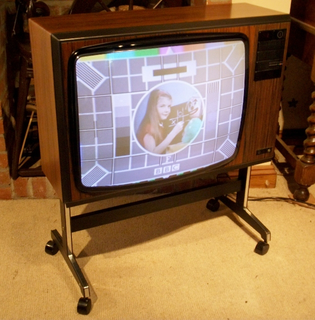The photograph captures a vintage 1970s-era TV with wood paneling on the sides, rectangular dials in the right-hand corner, and a sleek silver base equipped with caster wheels, enabling it to be easily moved around. This TV, likely positioned in front of a small brick fireplace, sits on a cream-colored carpet. The television is showing a BBC broadcast in color, characterized by a somewhat faded image displaying a countdown circle. In the center of the screen, there is a young girl, approximately nine years old, dressed in a red shirt, seemingly drawing tic-tac-toe lines while holding a small clown toy to her right. The background imagery on the TV screen features industrial patterns of rectangles and squares, complemented by a rainbow of yellow, blue, and green hues at the top. Behind the television, various objects, potentially another TV and shelves, as well as the TV's power cord, are faintly visible. The scene gives off a nostalgic, cozy atmosphere, emphasizing the retro element of the old-fashioned wheeled TV set.